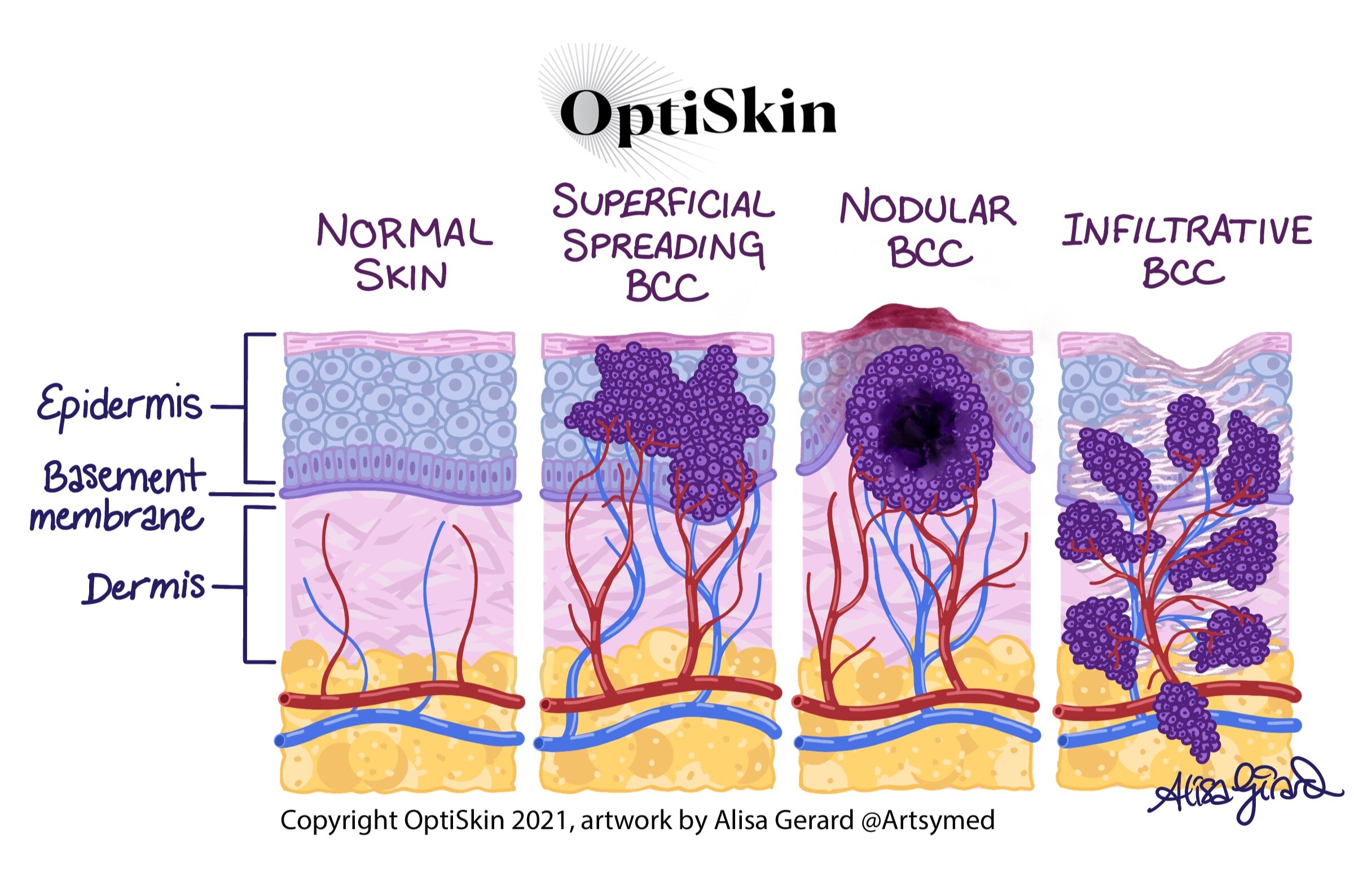This is a detailed cartoon-style infographic titled "OptiSkin," showcasing an anatomical cutaway view of various skin conditions. The illustration is divided into four columns, each depicting a different state of the skin, labeled in purple handwritten text at the top: "Normal Skin," "Superficial Spreading BCC," "Nodular BCC," and "Infiltrative BCC." Each column features a detailed diagram of skin layers, including the epidermis, basement membrane, and dermis, with labels indicating these sections. The colors used in the artwork are a harmonious mix of purples, pinks, yellows, reds, and blues. Blue and red veins or capillaries are depicted extending through the skin layers, and purple growths, resembling clusters of grapes, are seen forming under the skin in the diseased states. Attribution is given at the bottom left corner, where small black text reads "© OptiSkin 2021, Artwork by Alyssa Gerard at ArtsyMed." Alyssa Gerard's signature appears in purple at the bottom of the picture.